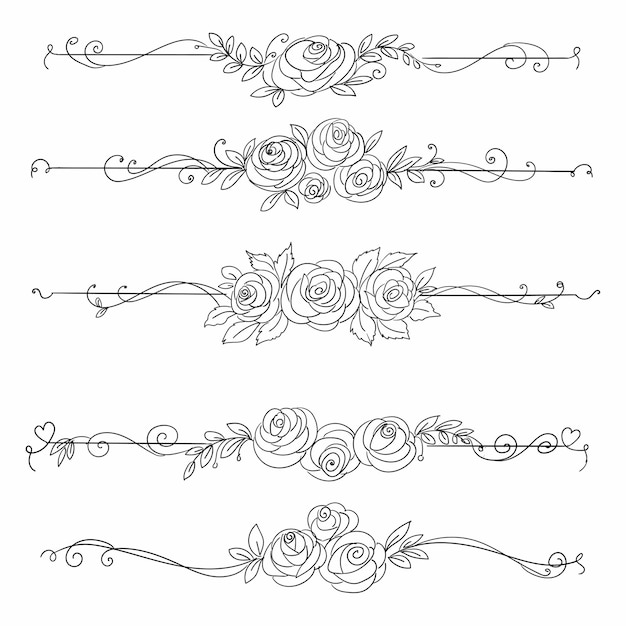The image contains five vertical black and white floral designs reminiscent of intricate, tattoo-style banners, each featuring different rose arrangements and linear elements in the background. At the top is a singular rose adorned with a few leaves and a long, thin stem branching out symmetrically. The second design showcases four roses—three larger ones and one smaller—interspersed with leaf motifs and extending lines. The third design features three evenly spaced roses in a straight line, surrounded by abundant leaves. The fourth design also has three roses, with the middle rose slightly lower than the other two, and its stems form a subtle heart shape at the bottom. The fifth and final design includes three roses, two larger flanking a smaller one, accompanied by swirling lines that curve towards the ends. Each banner is detailed with clear, delicate lines contributing to a cohesive and aesthetically pleasing floral pattern.